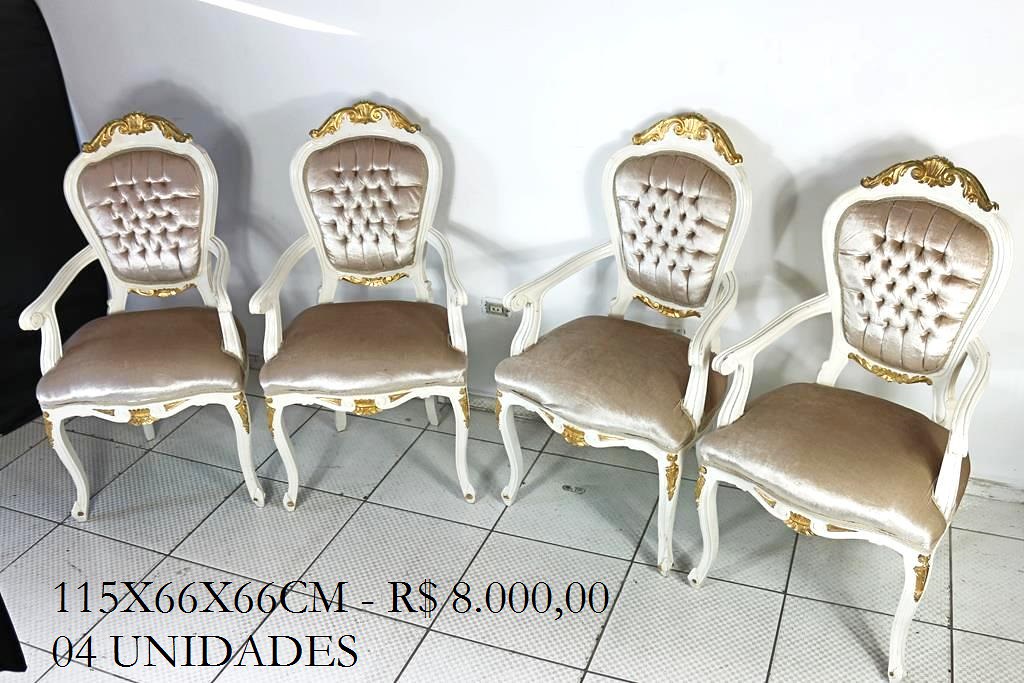The image showcases a set of four extravagant chairs placed side by side on a white ceramic-tiled floor. Each chair, reminiscent of royal antique furniture, is meticulously crafted, featuring a wooden frame painted in a creamy white hue adorned with opulent gold trim. The chairs boast luxurious, shiny, and silky beige cushions on both the seat and the button-tufted backrest, enhancing their regal appearance. The legs and arms of the chairs are intricately shaped with careful moulding and exhibit additional gold embellishments, especially on the front and sides. The background of the scene contrasts sharply, with a pure white wall and a black curtain on the left side of the frame. In the bottom left corner of the image, a label displays '115X66X66CM-R $8000' followed by '04 UNIDADES,' indicating specifics like dimensions and price.